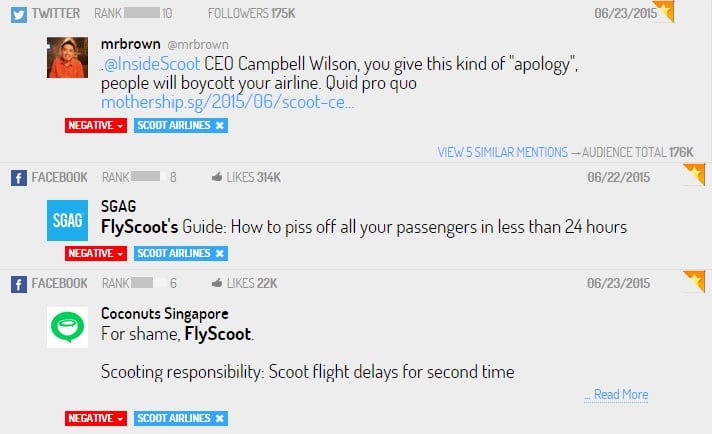Here's a more polished and detailed caption for the provided description:

---

A screenshot with a gray background features a comprehensive social media and news update concerning Scoot Airlines. At the top, Twitter statistics show a rank of 10, with @MrBrown garnering 175,000 followers as of June 23, 2015. An inset displays a picture of Mr. Brown along with his Twitter handle in blue, @InsideScoot, and a discussion involving CEO Campbell Wilson. The text suggests that an insincere apology could lead to a boycott of the airline.

Below, web content from mothership.sg dated June 2015 covers the topic, labeled "negative" in a red rectangle and "Scoot Airlines" in a blue rectangle with an 'X'.

The screenshot also includes an option to view five similar articles or mentors, totaling an audience of 176,000. Facebook analytics indicate a rank of 8, with 100 likes out of 314,000 as of June 22, 2015. 

Additional commentary from Sgag humorously refers to Scoot's potential misstep with the headline, "How to Piss Off All Your Passengers in Less than 24 Hours".

---

This polished version maintains all the details while structuring the information in a clearer and more coherent format.